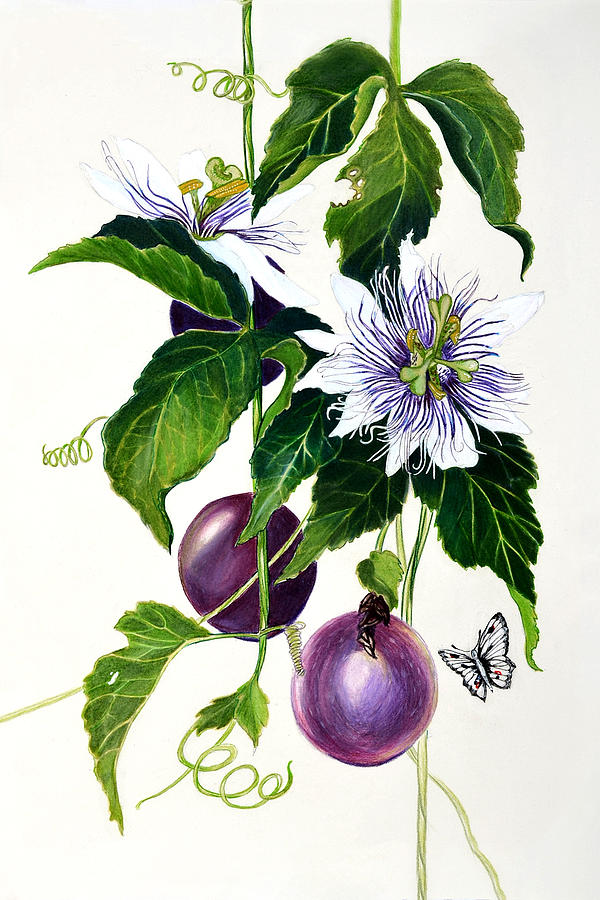The image depicts a highly detailed and elegant botanical drawing, likely from a book, of a grapevine with dark green leaves and flowing stems. The leaves are intricately detailed with lines and variations of lighter green shades, and one leaf shows a distinct bite mark. The background is a clean, cream color, highlighting the rich, dark hues of the plant. The vine bears white flowers with delicate purple striations and yellowish-green centers. Nearby, there are clusters of dark purple, almost metallic-looking grapes, indicating a variety of dark wine grapes. A butterfly, predominantly black and white with hints of red, is flying near the fruit, adding to the scene’s natural beauty. The image captures the plant in both flower and fruit stages, showcasing its full life cycle.